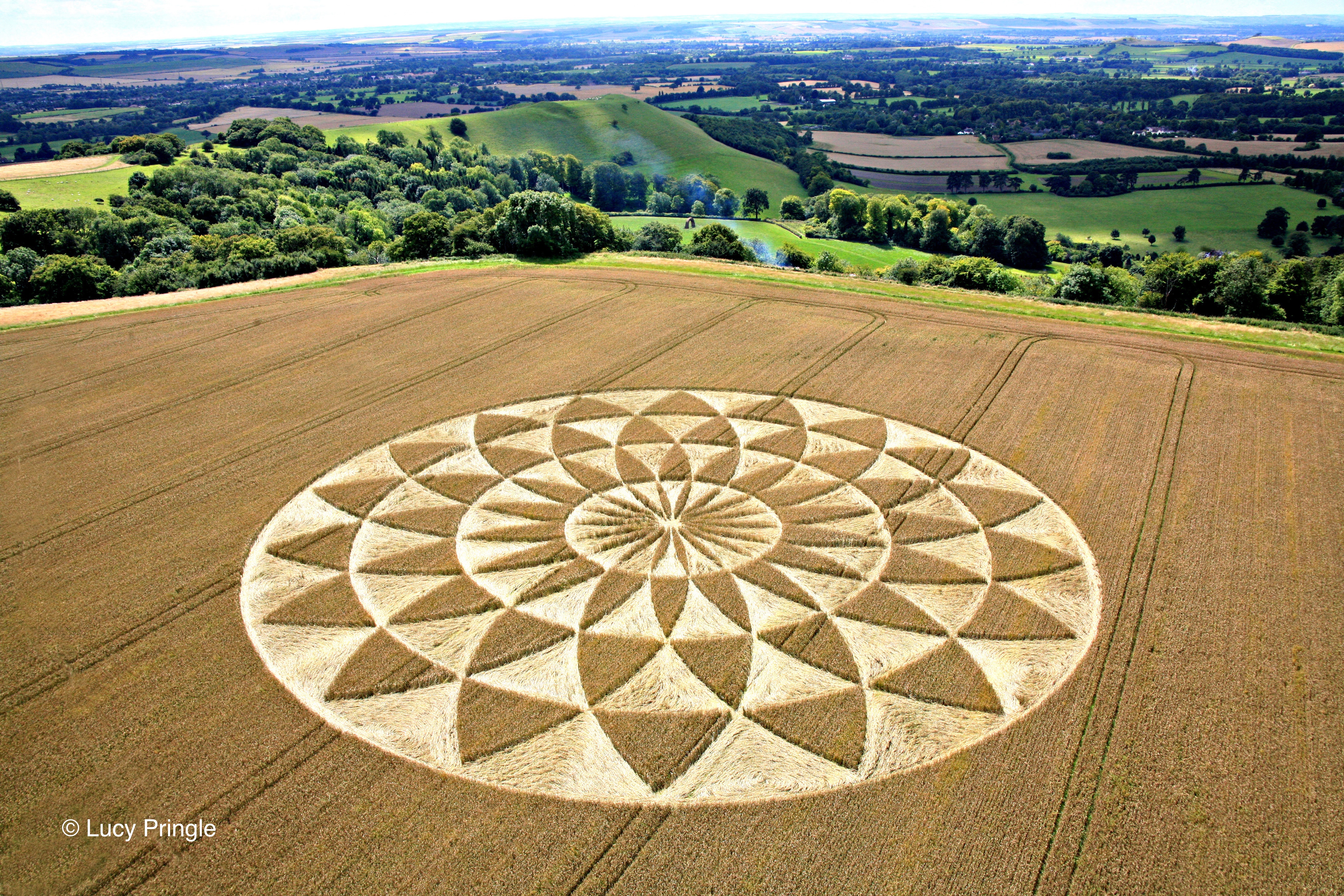This photograph, attributed to Lucy Pringle as watermarked in the bottom left corner, captures a stunning crop circle intricately carved into a plowed field. Dominating the bottom two-thirds of the image, the crop circle manifests a beautiful flower-like pattern with concentric rings emanating from the center, each intricately detailed with softly-shaped triangles that grow thinner towards the core, resembling spokes of a wheel. The crop itself is a pale, yellowy-beige hue, contrasting sharply with the darker hay color of the surrounding field. Beyond this mesmerizing design, the backdrop reveals a pastoral landscape featuring rolling hills adorned with rich, dark trees, additional fields stretching into the distance, and a few distant structures or houses. The image is striking in its precision and clarity, highlighting both the artistry of the crop circle and the serene rural environment encapsulating it.